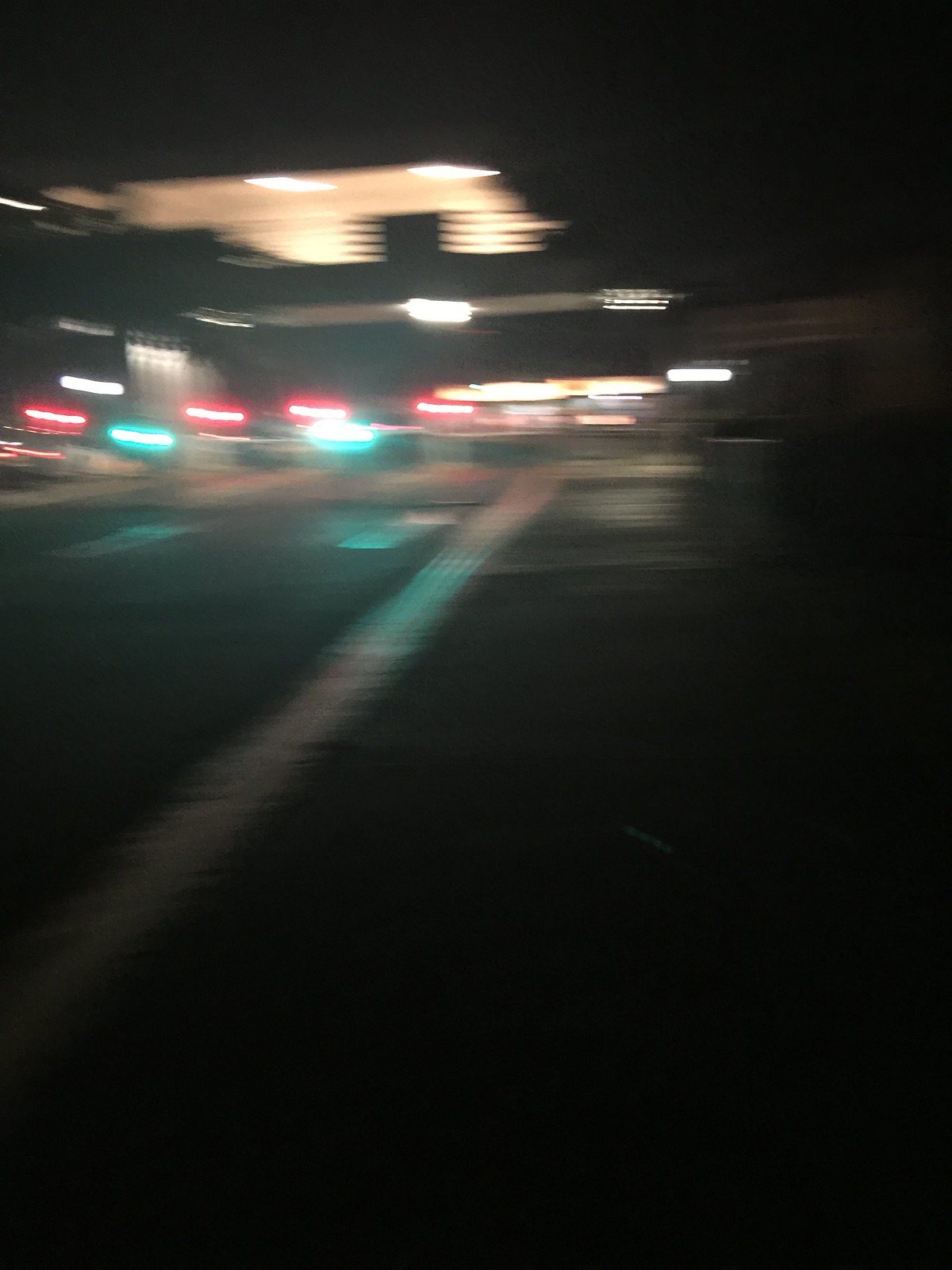The image captures a blurry and dark nighttime scene in portrait orientation, depicting an entryway that resembles a toll booth area or a parking lot. The photograph shows a series of green and red lights along different lanes, with motion blur suggesting the photographer was moving from left to right. In the background, there is a building that could be a help center or convenience store, which has multiple lights—red, light blue, yellow, and white—illuminating its structure. The ground is dark gray asphalt, featuring white lines that indicate lane edges, and resembles a crosswalk. The scene is dominated by various lights, with red and green lights forming distinct rows, set against a pitch-black night sky.